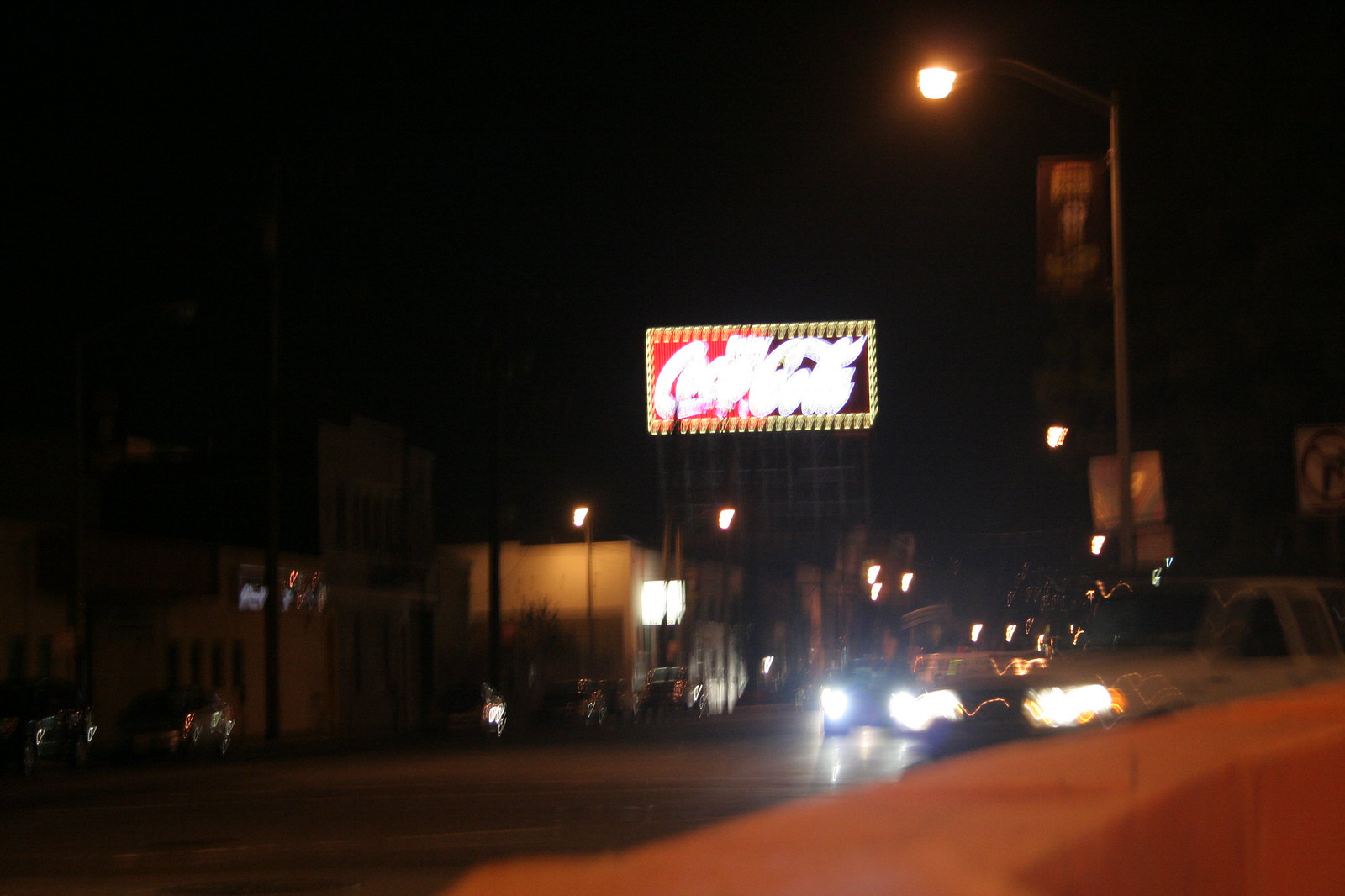The photograph depicts an interior view of a car in motion at night, identifiable by the visibility of the dashboard. The windshield is prominently marked with dirt and specks, which are clearly illuminated by the ambient light. There's a noticeable glare on the image, indicative of the flash or reflection from the picture-taking process. In the distance, a red sign bordered with lights reads, "Enjoy Coca-Cola," although the word "enjoy" appears considerably blurred, while "Coca-Cola" is slightly more discernible. Several cars with their headlights on are visible in the foreground, contributing to the nocturnal atmosphere of the scene.